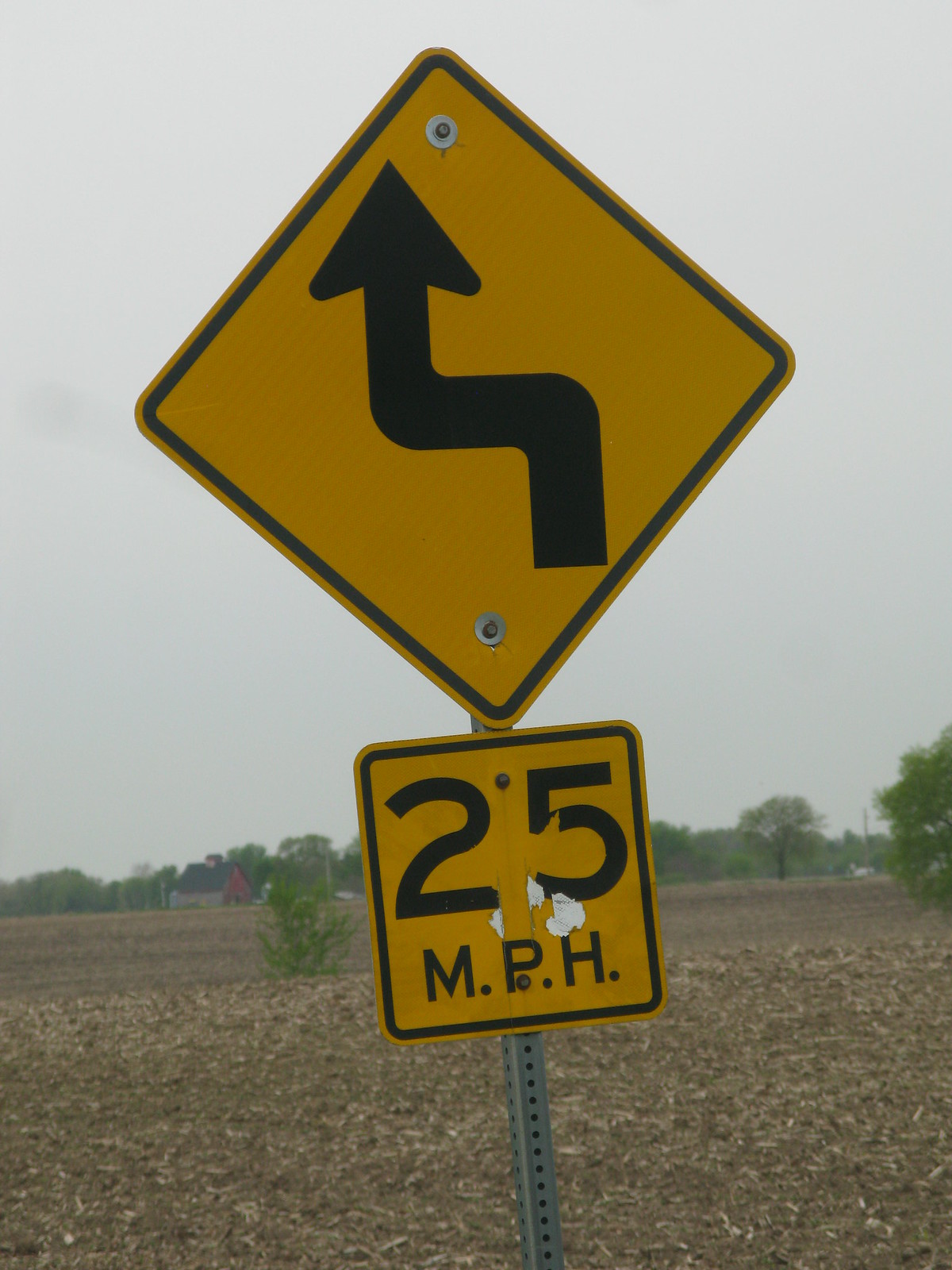This photograph captures a rural setting characterized by a large plowed field stretching out under an overcast sky, evoking a sense of the outskirts or countryside. The focal point of the image is a prominent road sign positioned in the foreground. The sign consists of two parts: a yellow triangular top section with a black winding arrow indicating a curvy road ahead, and a yellow square section below displaying "25 MPH" in black print. The signpost is made of steel and features holes, suggesting wear and exposure to the elements. Surrounding the field in the distance are sparse trees, adding to the rural ambiance. A notable feature in the background includes a red house or barn with a blue sloped roof, contributing to the farmland aesthetic. The sign itself shows signs of age, with some rust and metal showing through, indicative of the passage of time and the outdoor environment.